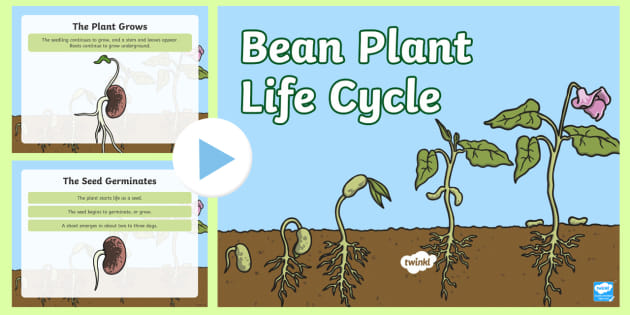The image shows a detailed cartoon diagram of the bean plant life cycle, appearing as a screenshot of a video with a play button in the center—a white circle with a blue triangle. The background is light blue with the title "Bean Plant Life Cycle" in white text bordered in green. The life cycle is depicted in five stages on the right side: starting with a bean seed sprouting with a small root, then a sprout emerging above the soil with extensive roots, followed by a growing stem and initial leaves, progressing to a larger plant with more leaves, and finally reaching full growth with three large leaves and a pinkish flower. The left side features two smaller sections: one at the top left labeled "The Plant Grows," and another at the bottom left labeled "The Seed Germinates," providing detailed information about each process. The overall image is colorful, bright, and clearly illustrated, making the stages and details easy to see.